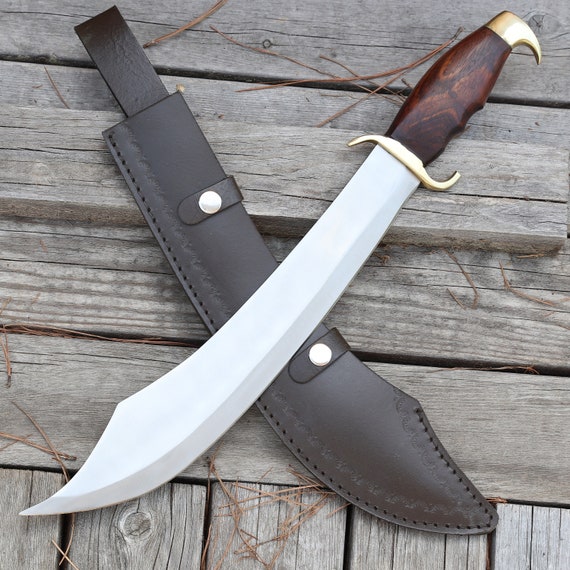The photograph features a large, Bowie-like knife with a dark, stained wooden handle situated in the upper right corner of the image, extending diagonally across the frame to the lower left. The handle end has a gold thorn or animal claw-like design, and there is a gold cross-guard separating it from the blade. The blade itself is broad, curved, and reminiscent of a scimitar. This knife rests atop a dark brown leather sheath, which has a belt loop and small snap buttons. The sheath extends diagonally from the upper left to the lower right, creating an X shape with the knife. Both items are placed on a weathered, gray, rustic wooden deck scattered with a few long brown pine needles. The overall scene exudes a sense of rustic elegance, combining elements of natural wood textures with the knife's intricate design and metallic accents.